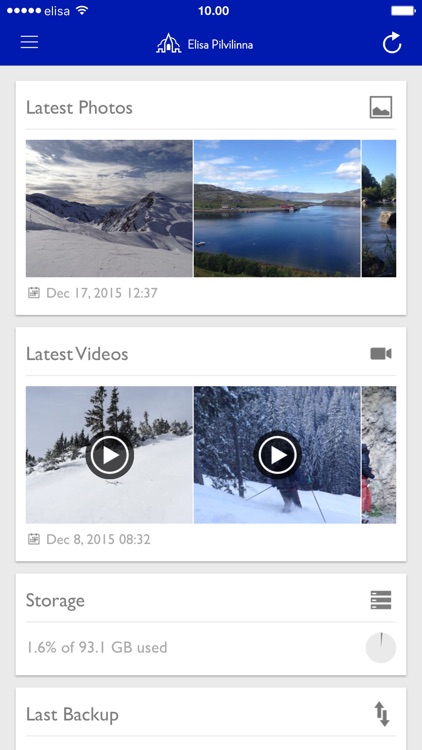In this image, we see the interface of a cell phone app displaying various media files and information. At the top left, there are five white dots, the name "Eliza," and a Wi-Fi icon. On the right-hand side, the battery bar is full, and the time is displayed at the center, reading 10:00. Below that, on the left, there are three horizontal lines indicating a tab menu, followed by the name "Eliza P." To the right, there is a refresh icon. The background color of this section is blue.

The first section below this header is labeled "Latest Photos." It shows two complete photos and a partial view of a third. The timestamp for these photos is December 17, 2015, at 12:37. The next section below is titled "Latest Videos," displaying two full videos and a portion of a third. These videos are timestamped December 8, 2015, at 08:32.

Further down, there is a section labeled "Storage," indicating that 1.6% of 93.1 GB has been used. Below that, another section is labeled "Last Backup." The background between each section is light gray, and there are narrow columns of this light gray color running vertically along the left and right sides of the image.